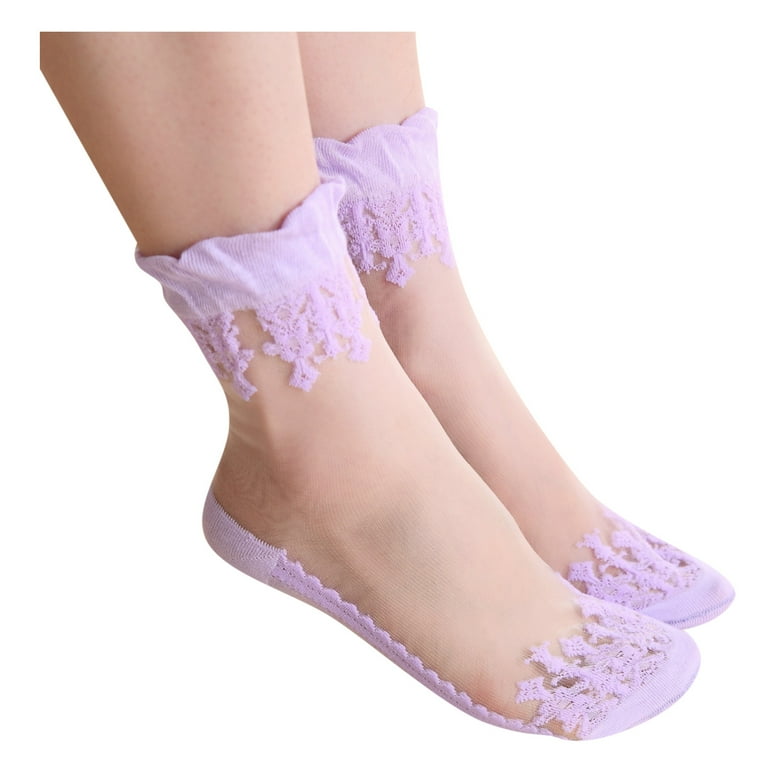This photo features the bottom half of a woman's legs from the shins down, showcasing her feet adorned in sheer, translucent socks set against a white background. The socks, crafted from a nearly transparent nylon-like material, create the illusion of bare skin on the top and sides of the foot. Adorned with a delicate lavender hue, the socks boast intricate details: a lace border extends from the heel to the toe, highlighting floral embroidery on both the toe area and the bottom of the feet. Above the ankle, the socks feature an embroidered, ruffled rim adding a touch of elegance to the design. The woman's feet, positioned side by side with toes pointing to the right, are the focal point of the image, emphasizing the intricate craftsmanship of the lace and embroidery work that enhances the sheer fabric of the socks.